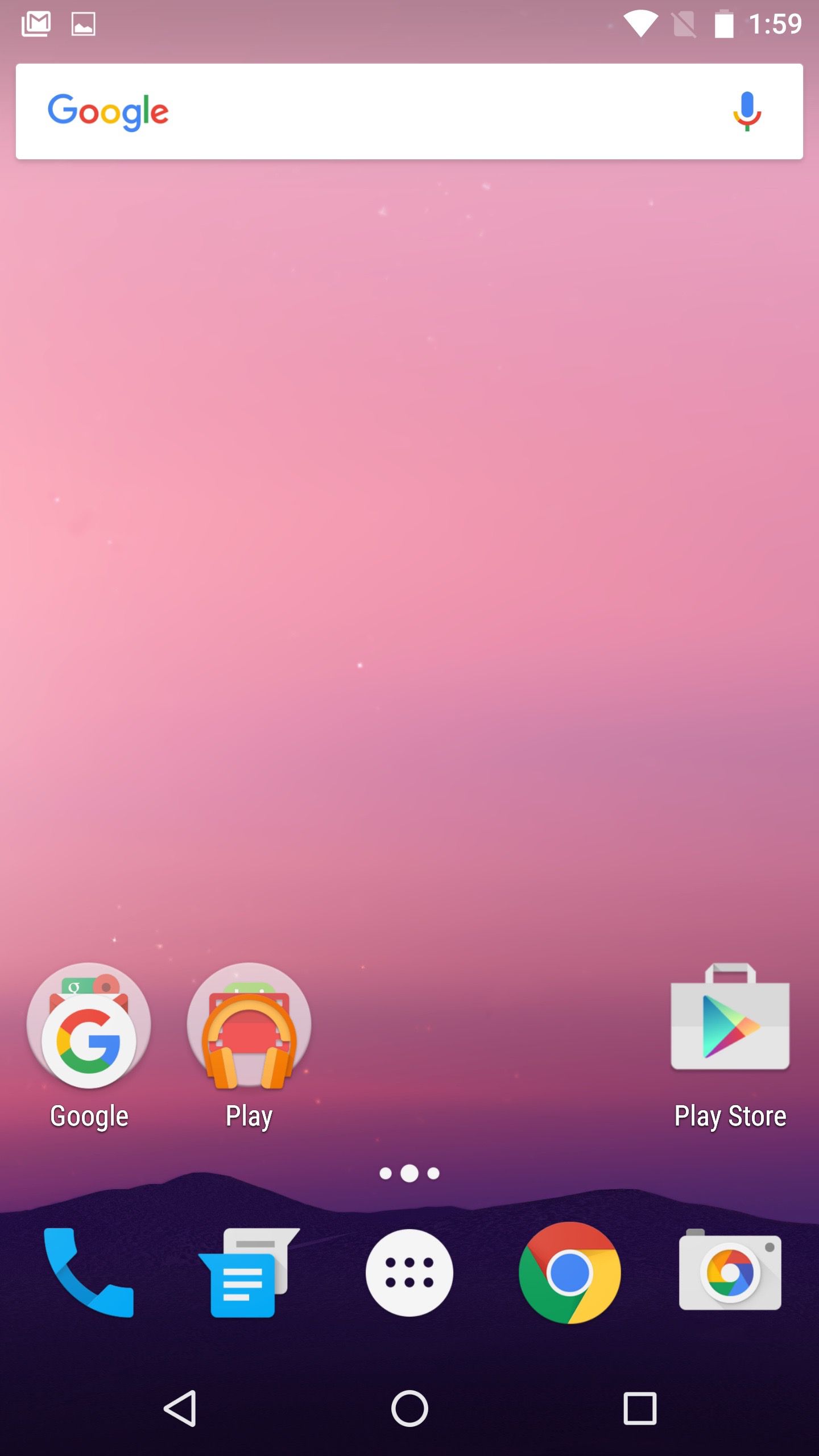In this image, we observe a detailed screenshot from a mobile device. In the upper left corner, icons for Gmail, Photos, and Images are clearly visible. On the upper right corner, the Wi-Fi signal is active, the battery is fully charged, and the time displayed is 1:59. The wallpaper showcases a beautiful aesthetic with a muted pink background featuring a silhouette of a dark mountain at the bottom.

At the center, a Google search box with a microphone icon is prominent. Below the search box, from left to right, there's a Google icon. Right behind it, the outline of the Gmail icon in a pink circle is visible. Further right, there’s a circle housing a pair of yellow and orange headphones, and underneath, in gray text, it reads "Play."

To the extreme right side, the Play Store icon is noticeable. Lining the bottom of the screen are icons for various applications: a blue telephone icon, an icon representing two stacked sheets of paper or text, the Google Chrome browser icon, and a camera icon.